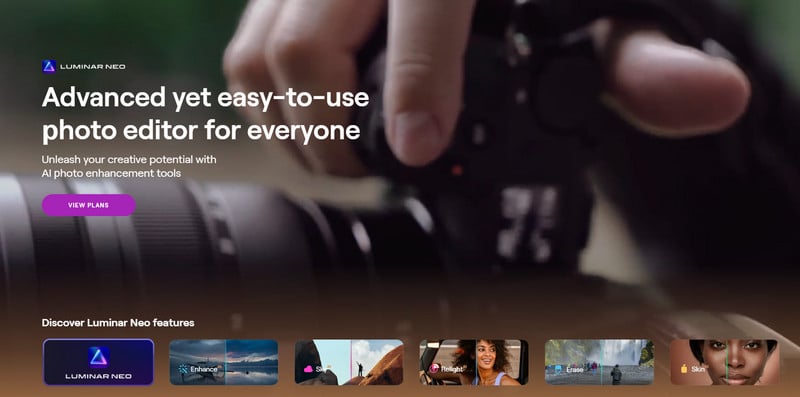A narrow horizontal rectangular advertisement prominently displays a hand holding a DSLR camera with a large zoom lens against a dark background. Positioned in the upper left corner, the blue Luminar Neo logo is clearly visible. Below the logo, white text reads: "Advanced yet easy to use photo editor for everyone," followed by "Unleash your creative potential with AI photo enhancement tools." Toward the bottom, a purple rectangle invites viewers to "View Plans," suggesting different pricing options. Below this, the text "Discover Luminar Neo features" is displayed above several smaller images showcasing the software's capabilities, such as color correction and various filters, presented with before and after comparisons.